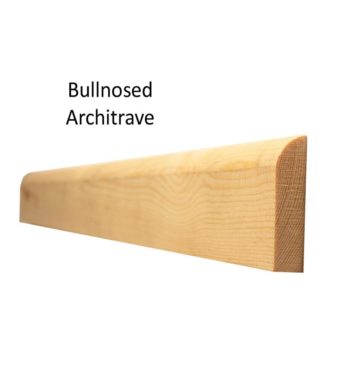This image depicts a rectangular piece of wood, identified as a Bull-Nosed Architrave, set at an angle. The wood, a brown material resembling plywood with visible grain, features a distinctive rounded top or arched upper edge. The sides of the wood piece are angular and straight, and the bottom is flat, enabling it to fit snugly against a flat surface like a wall. The perspective in the image shows the wood appearing larger on the right side and tapering off to the left, giving a sense of depth. Notably, the lighting causes the wood to appear darker as it recedes into the background. Displayed over the top left of the image is the text “Bull-Nosed Architrave” in black, standard font, akin to Calibri. The architrave is likely a molding used along the base of a wall, with its rounded top edge adding a subtle yet refined detail.